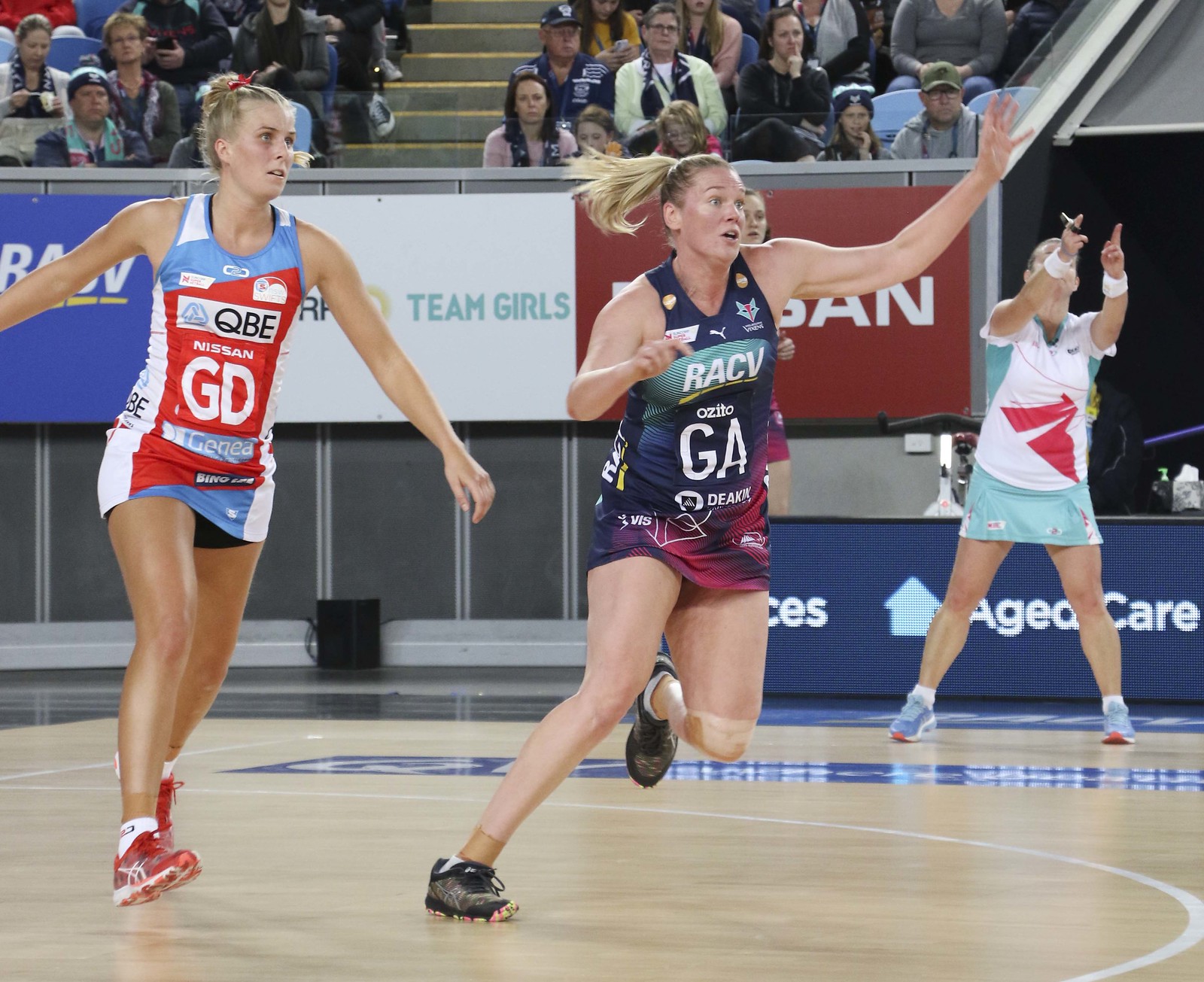The color photograph, taken from inside a stadium or arena, captures a close-up shot of two tall young women engaged in a sport on a polished wooden court. Both women have blonde hair pulled up into ponytails and are wearing different uniforms, indicating they are on different teams. The girl on the left sports a red, white, and blue uniform with "QBE Nissan GD" emblazoned on the front, complemented by red shoes. Meanwhile, the girl on the right dons a dark blue and purple uniform bearing the letters "R-A-C-Y-G-A," paired with black shoes. They both seem to be intently focused on something above them. Behind them, seated on the steps or bleacher seats, is a crowd of spectators, some of whom are gesturing animatedly. Notably, a woman on the far right in a pale blue skirt and a blue and white top has her fingers pointed in the air. This crowded arena, adorned with banners in blue, white, and red, sets the stage for what appears to be an uncertain sport, though the floor suggests it might be a basketball court. The unusual attire, which includes skorts, further adds to the ambiguity of the sport being played.